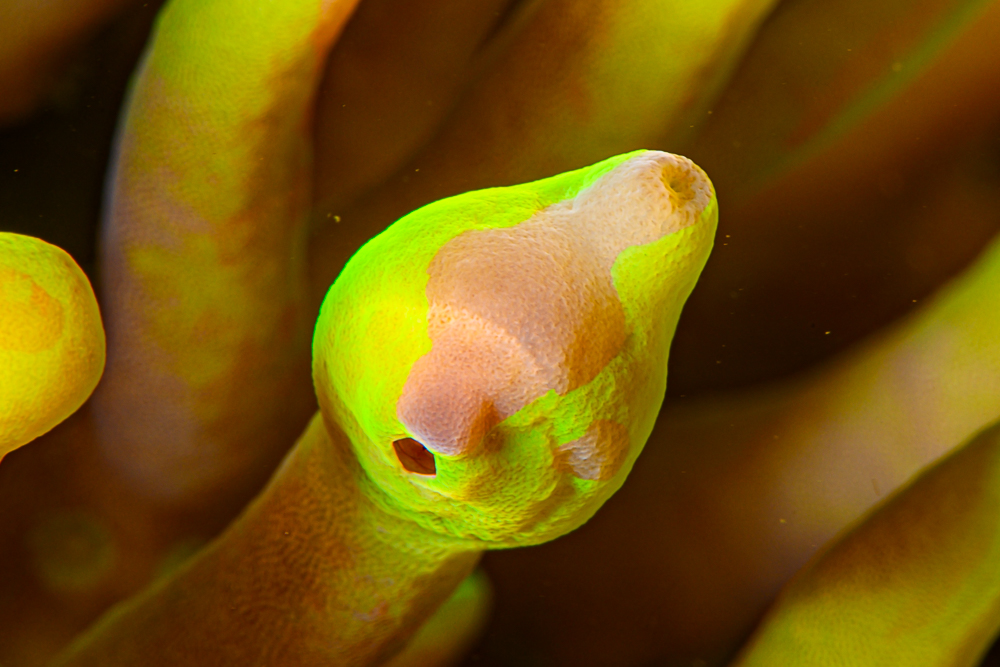This detailed close-up image captures a mysterious underwater scene, likely within a large aquarium or fish tank environment. Centered in the image is a curious yellowish, tube-like structure resembling a plant or sea life form. The stalk emerges from the base, culminating in a bulbous, rounded head adorned with intricate patterns. The head features varying hues, including a pinkish or light brown area with two prominent holes. One hole, smaller and within the patterned region, contrasts with the larger hole situated outside this design. The play of light creates a slight glow, highlighting the neon yellow coloration and the peach-like blotches on the bulb. Surrounding the central bulb, similar structures are partially visible, suggesting this is part of a larger cluster of such organisms. The background appears darker, enhancing the clarity and vibrant detail of the foreground subject, which exudes an almost otherworldly, biological charm.